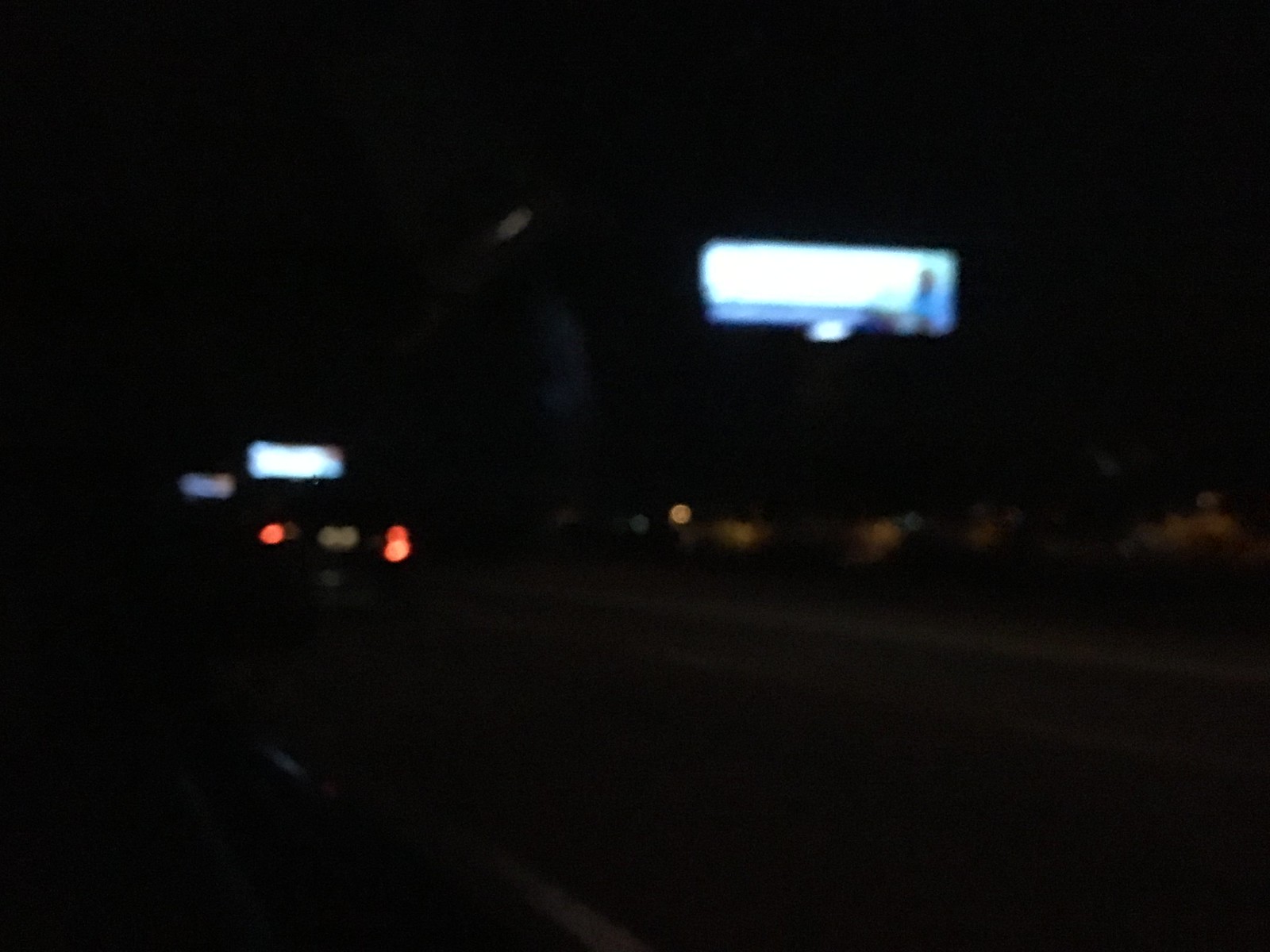In this moderately blurry nighttime photograph, it appears to have been taken from the perspective of a passenger in a moving vehicle on a highway. The image is very dark and taken in motion, resulting in poor quality. The scene shows a stretch of road with faint white road markings visible on the pavement, including a solid white line and a dotted center line. At the center of the image is another car, recognizable by its two red taillights and a reflective license plate underneath. On top of this car, there is a bright white object that suggests it might be a taxi. In the background, three illuminated billboards can be seen, one being quite large while the other two are smaller. Due to the blurriness, details about the person with a blue shirt on one of the billboards are indistinct. The overall darkness and blurriness of the image make it difficult to distinguish precise details.